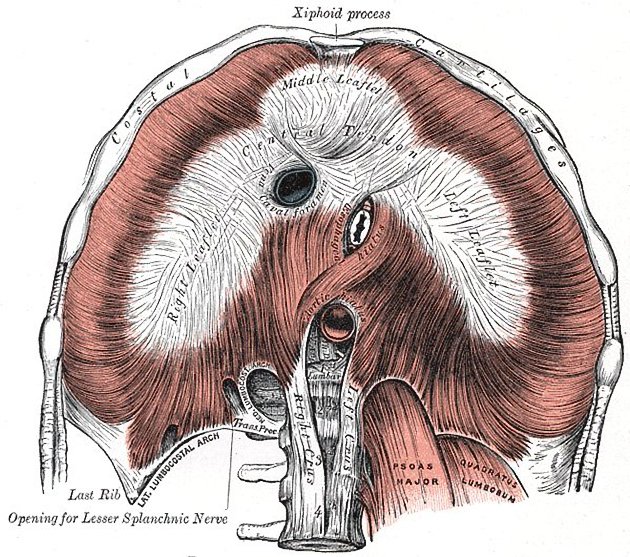The illustration appears to be a detailed anatomical drawing from a medical textbook, showcasing part of the thoracic region. Dominated by a palette of copper brown, gray, and white reminiscent of Escher's work, the image highlights various components of the rib cage and diaphragm. At the top of the image is the xiphoid process, while a white border labeled "costal cartilages" surrounds the entire illustration.

Central to the image is a dome-shaped structure, depicted in a red textured circular area, marked by an arrangement resembling a heart made from skeins of yarn. Inside this formation are further intertwined white skeins. The diagram identifies several key elements, including the middle leaflet, central tendon, right leaflet, and left leaflet. These anatomical features appear to converge toward an area that abruptly ends, suggesting the representation of a bone or cartilage segment whose labels are not entirely readable.

The lower-left corner of the image provides a specific annotation for the "last rib opening for lesser splanchnic nerve," hinting at the detailed nerve innervation in this section. Despite some ambiguity in label clarity, the overall detailed annotations—ranging from the xiphoid process and costal cartilages to various leaflets and tendon structures—imply a thorough depiction of the thoracic anatomy, likely intended for educational purposes in medical literature.